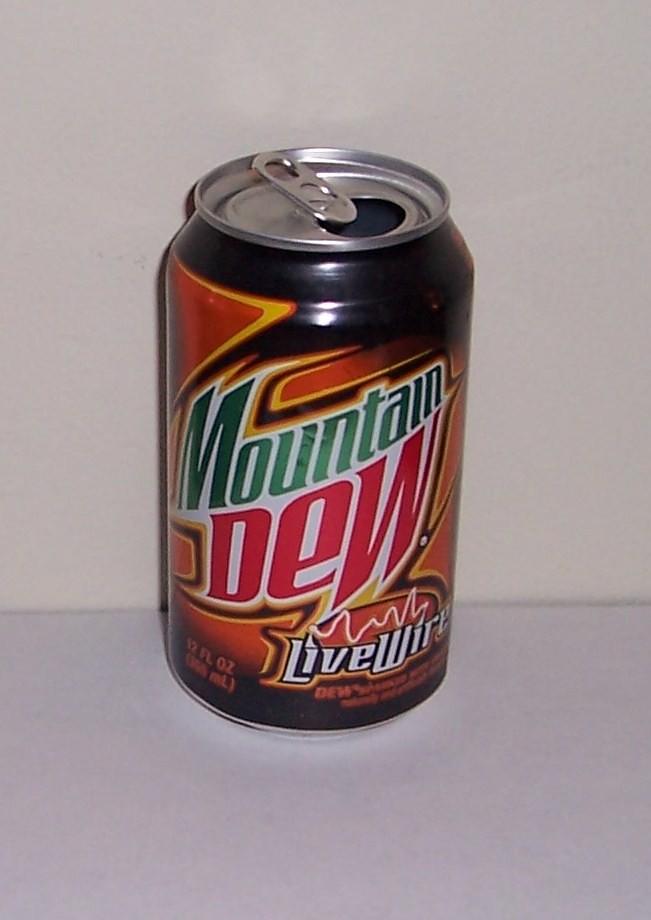The image features an open can of Mountain Dew Live Wire prominently displayed against a white floor and wall, providing a sharp contrast that highlights the can's vibrant design. The can itself predominantly showcases a dynamic mix of colors, with a striking black base accented by an orange glow that adds depth to its appearance. The iconic "Mountain Dew" logo stands out, with the word "Mountain" slanted towards the top right in a bold green, while "Dew" is larger, featuring a distinctive red hue with a prominent, oversized 'W'. The logo is set against a white background, bordered by an energetic blend of yellow, black, and orange.

Below the main logo, the words "Live Wire" are displayed in white text outlined in black, accompanied by a small squiggly, wire-like graphic that adds a unique touch, connecting two points above the name. Further down, the can indicates its volume, "12 FL OZ," in small white text positioned at the bottom left. Additionally, there is some descriptive text in orange beneath the "Live Wire" label. The silver top of the can is visible with the typical opening hole, emphasizing that the can has been opened. The overall composition of the image captures the energetic and dynamic essence of Mountain Dew Live Wire, with its vibrant colors and engaging design.